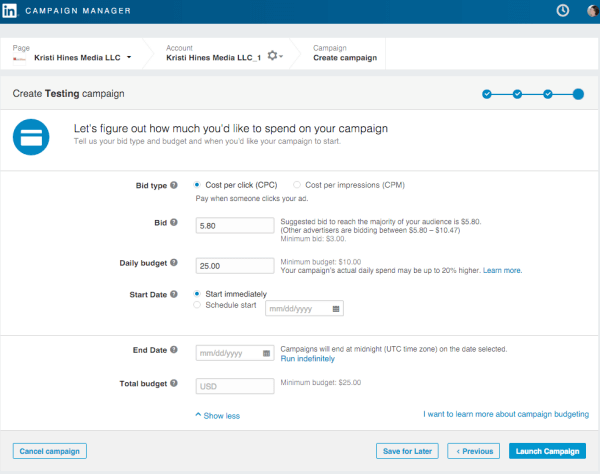**Detailed Caption:**

This screenshot depicts a campaign setup page on the LinkedIn website, specifically tailored for a user from Christy Hines Media LLC. The campaign manager is on the third step of a four-step process. The progress is indicated by checkmarks next to the first three steps.

The page invites the user to create a "Testing Campaign," with the word "testing" emphasized in bold. Here, users are asked to specify their bid type, budget, and campaign start date. Available bid types include Cost Per Click (CPC) and Cost Per Impression (CPM), with an example bid set at $5.80. The daily budget is listed as $25.

Under the campaign scheduling options, "Start Immediately" is selected by default, with an option to set a custom start date or let the campaign run indefinitely. The end date field is empty, but there's a note stating that campaigns will end at midnight UTC if no date is specified. 

The page also features a text box for entering the total budget, which currently shows a minimum budget requirement of $25 but is left blank.

Additional functionality includes an expandable section that can be minimized with a "show less" button. At the very bottom of the page, users can cancel the campaign with a provided link. On the bottom right, there are three clickable options: "Save for Later," "Previous," and "Launch Campaign," the latter highlighted with a blue outline.